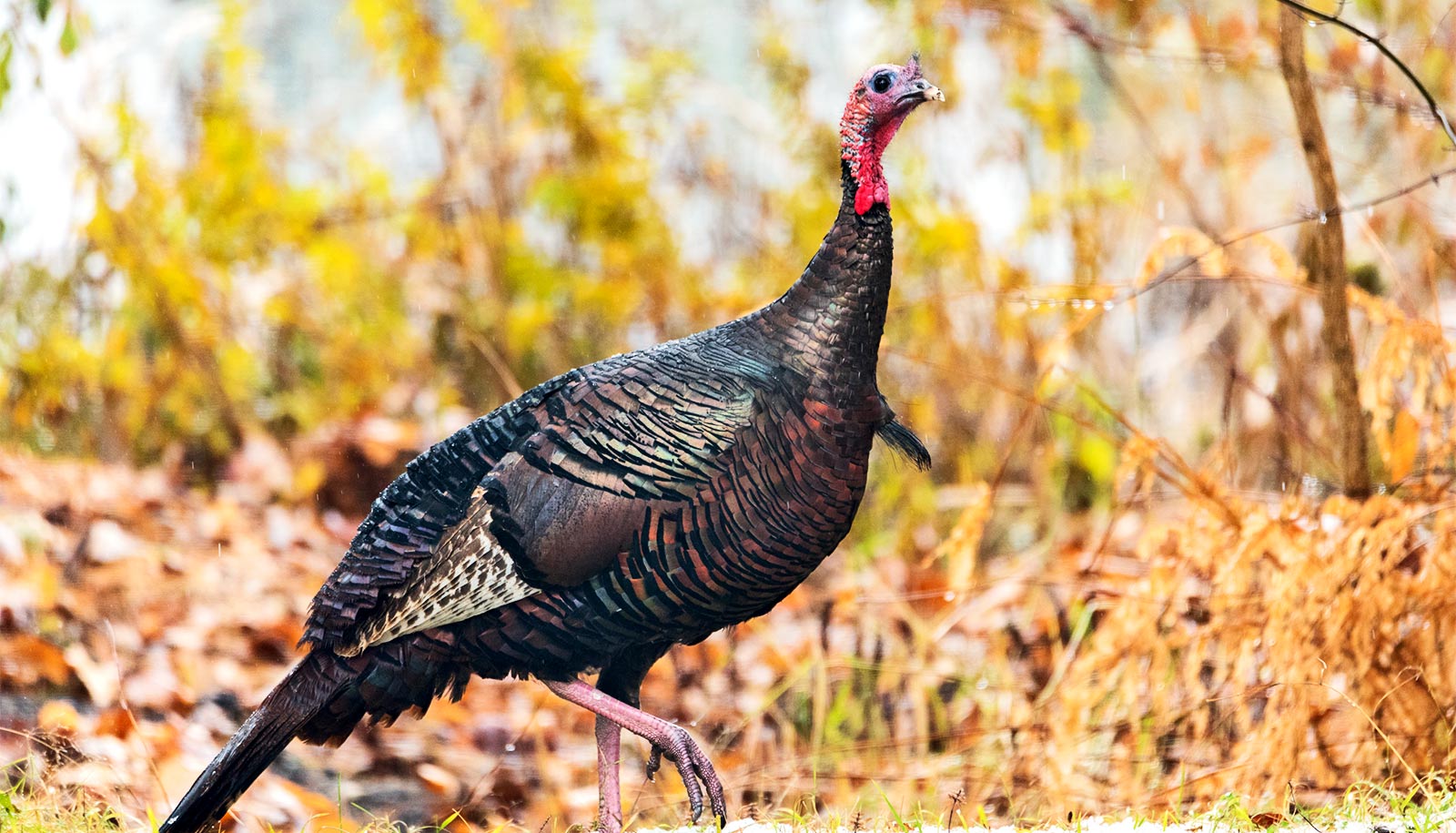In the image, a wild turkey walks through a fall landscape, displaying iridescent green and red feathers with a scaly texture. The turkey's face and neck are red, with a beady eye and dark tail feathers. It’s in mid-stride, one foot planted while the other is lifted. Its pinkish, scaly feet add to its dinosaur-like appearance. Surrounding the turkey are yellowing leaves on trees, various shades of brown and green foliage, and a backdrop of blurred brush and shrub stems, emphasizing the autumn setting. The turkey's unusual feather pattern and overall large size, likely around 10-15 pounds, help it blend into the fall foliage.